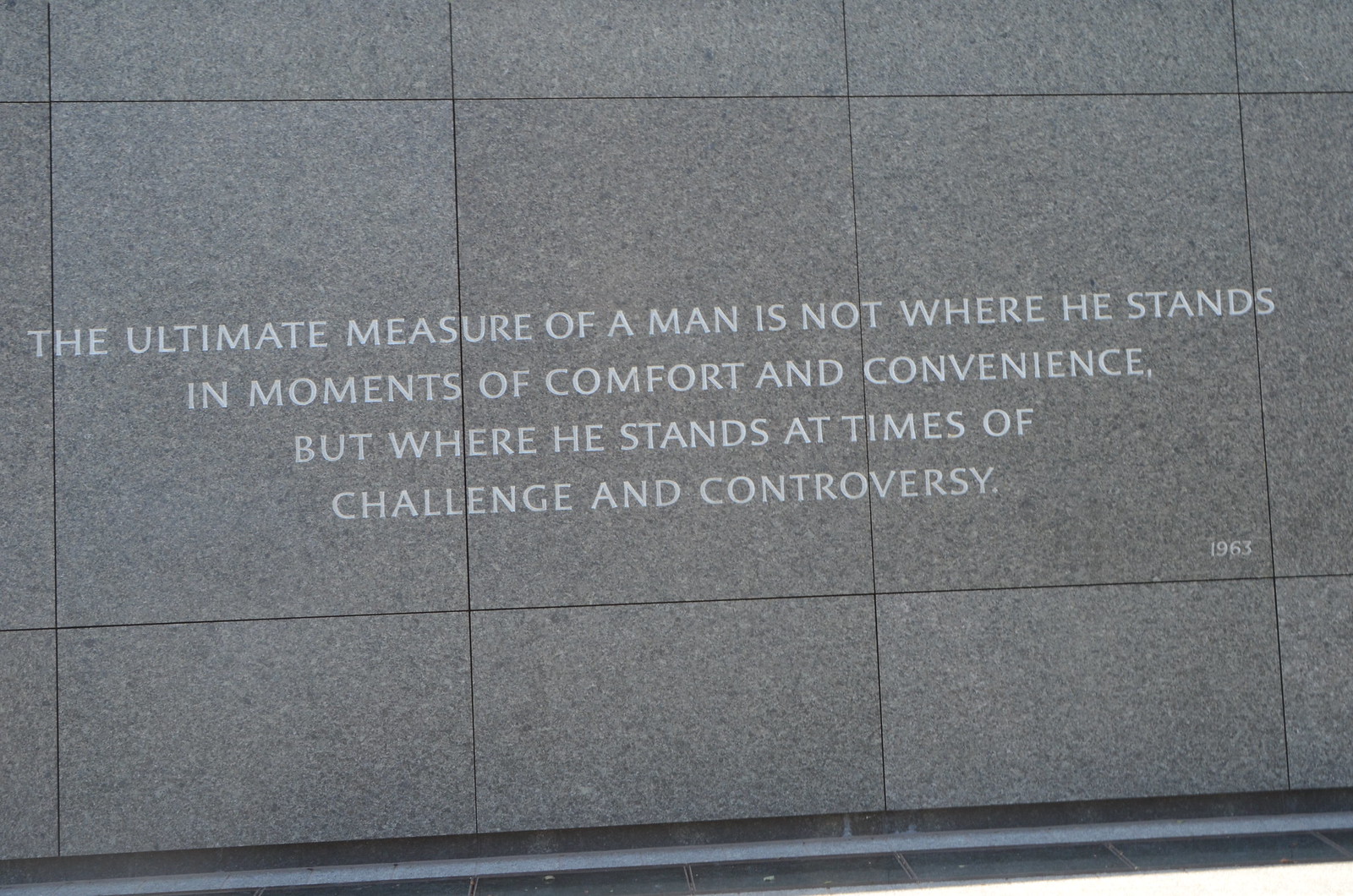The photo captures a solemn, gray memorial wall composed of large, smooth marble squares. At the center, inscribed in striking white letters, is the quote: "The ultimate measure of a man is not where he stands in moments of comfort and convenience, but where he stands at times of challenge and controversy." The surrounding squares are smaller, accentuating the central text. In the lower right-hand corner of the inscribed square, the year "1963" is etched. The wall stands alone, void of any other objects, emphasizing its stark and contemplative nature.